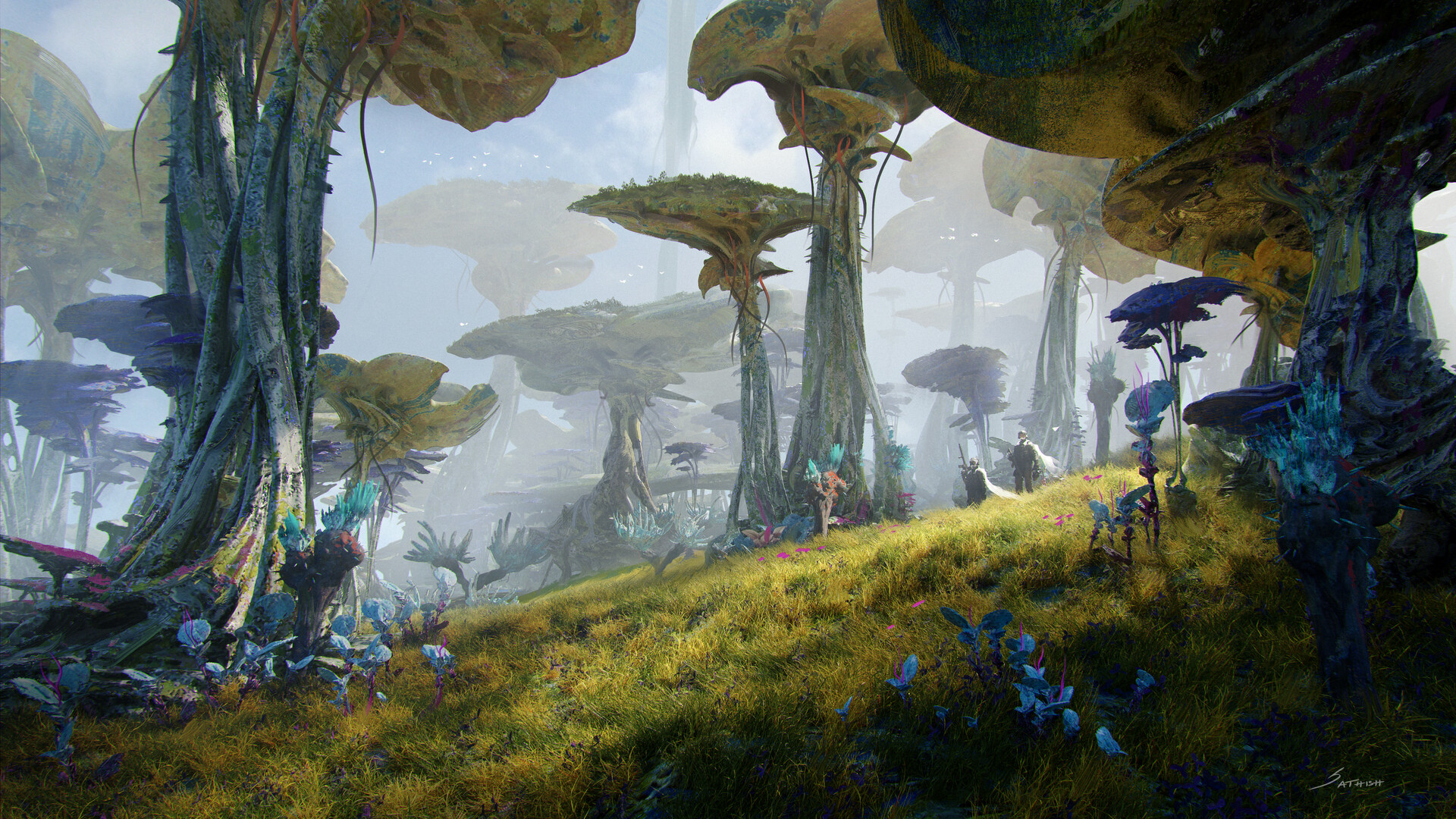In this highly detailed digital painting, reminiscent of a fantasy video game or an artist's rendition of a fictional universe, we are transported to an otherworldly landscape. The scene is dominated by enormous, tree-like structures with whitish-beige trunks that tower into the sky, terminating in flat, mushroom-shaped tops. These unusual formations are dispersed across grassy hills that slope gently. The overall color palette is a blend of blue, green, teal, and purple tints, contributing to the alien atmosphere. In the distance, barely discernible figures wearing helmets and possibly capes stand with one of them holding what appears to be a weapon. The sky overhead is a hazy blue, adding to the mysterious and futuristic ambiance. Towards the very back of the landscape, a colossal structure, seemingly man-made or alien-crafted, rises prominently. Adding a final touch of authenticity, the artist's signature adorns the bottom right-hand corner of the canvas.